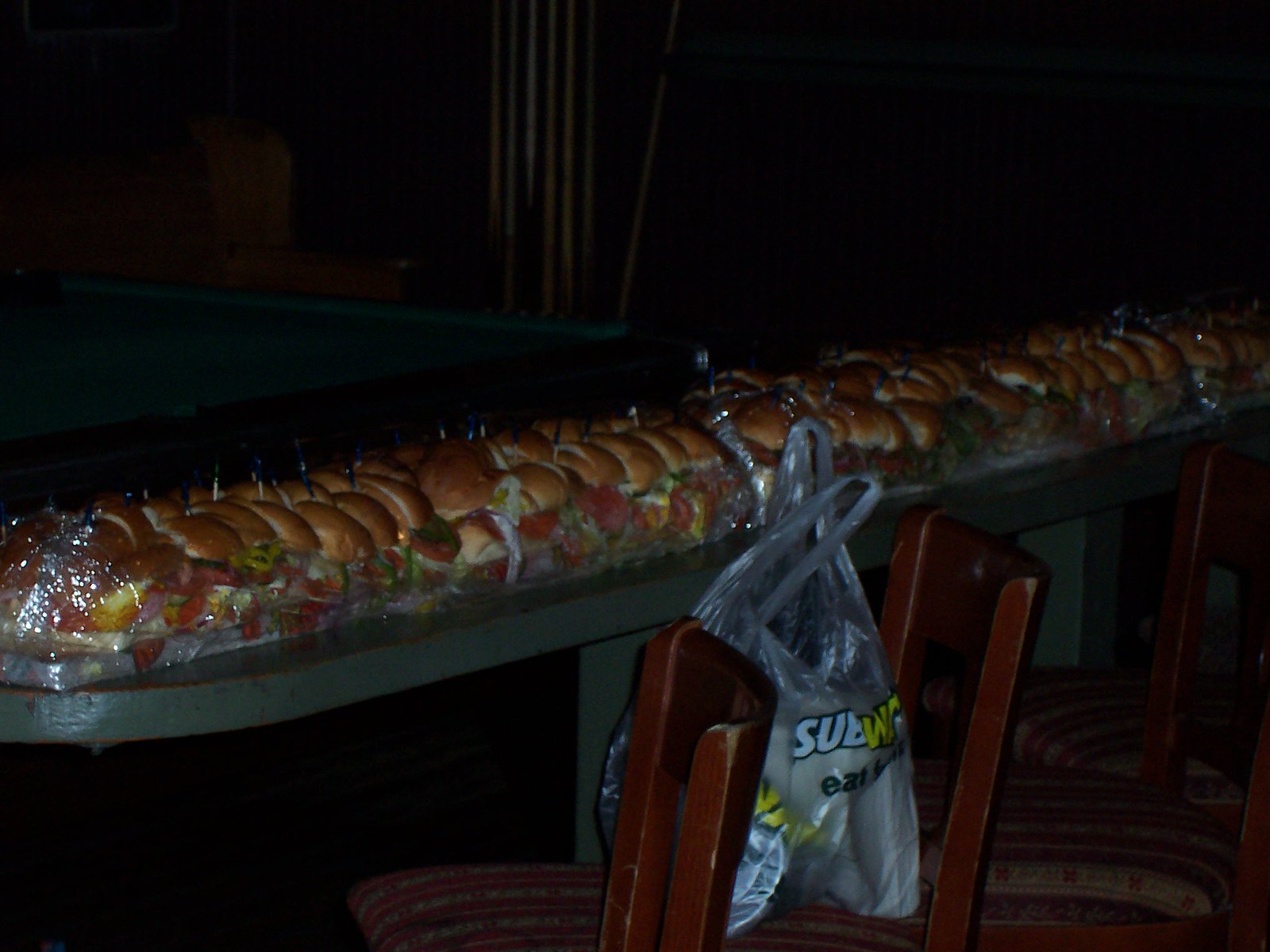This photograph captures a dimly lit room, possibly taken at night, showcasing a preparation setup for a catering event or party featuring Subway sandwiches. Dominating the image is a lengthy table that appears to be either green or gray, extending diagonally from the lower left to the upper right frame. The table is densely covered with a long stretch of subs, creating the appearance of one gigantic sandwich segmented into smaller pieces. Each piece is pre-cut and adorned with toothpicks topped with small blue foils. The sandwiches reveal fillings of lettuce, tomatoes, and possibly banana peppers, though the exact contents are somewhat obscured by the lighting.

In the foreground, there are several well-worn wooden chairs with red and tan striped cushions featuring floral patterns. Among these, one chair prominently holds a clear plastic Subway bag branded with the Subway logo and the slogan "Eat Fresh." The bag appears to contain additional items, though their specifics are indeterminate. The background is enveloped in darkness, making it difficult to discern further details, but faint outlines suggest additional structures, potentially including a pool table and cue sticks, indicating a recreational setting such as a den or playroom.